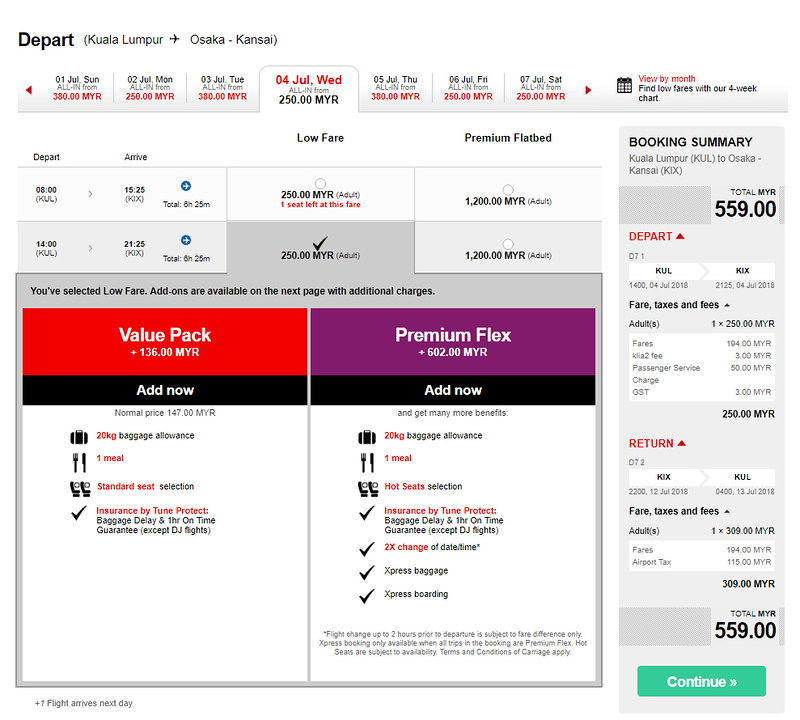This image showcases a flight booking interface for a trip from Kuala Lumpur (KUL) to Osaka (KIX), specifically highlighting the departure options available for Wednesday, July 4th. The details provided include various fare types, add-ons, and a booking summary. 

**Departure Options:**
- **Average Seating Capacity:** 120 MYR
- **Selected Fare Types:**
  - *Low Fare:* 250 MYR
  - *Premium Flatbed:* 1200 MYR

**Add-ons:**
- *Value Pack (Additional 136 MYR):* 
  - 20 kg baggage allowance 
  - 1 meal 
  - Standard seat selection 
  - Insurance by TuneProtect (includes baggage delay and on-time guarantee, except DJ flights)
- *Premium Flex (Additional 602 MYR):* 
  - 20 kg baggage allowance 
  - 1 meal 
  - Hot seats selection 
  - Insurance by TuneProtect (includes baggage delay and on-time guarantee, except DJ flights)
  - Two-time change of date and/or time 
  - Express baggage 
  - Express boarding

**Booking Summary:**
- Total: 559 MYR
- **KUL to KIX:**
  - Departure Date: July 4th, 2018
  - Flight: D71
  - Time: 14:00 to 21:25
  - Breakdown of Fare, Taxes, and Fees:
    - Fare: 194 MYR
    - Kila 2 Passenger Service Charge: 30 MYR
    - GST: 12 MYR
    - Total: 250 MYR
- **KIX to KUL:**
  - Return Date: July 14th, 2018
  - Flight: D72
  - Time: 22:00 to 06:00
  - Breakdown of Fare, Taxes, and Fees:
    - Fare: 309 MYR
    - Airport Tax: 0
    - Total: 309 MYR

The interface provides options to continue and offers a choice between a lower fare with fewer benefits or a premium fare with additional perks, allowing flexibility based on the traveler's preference and budget.